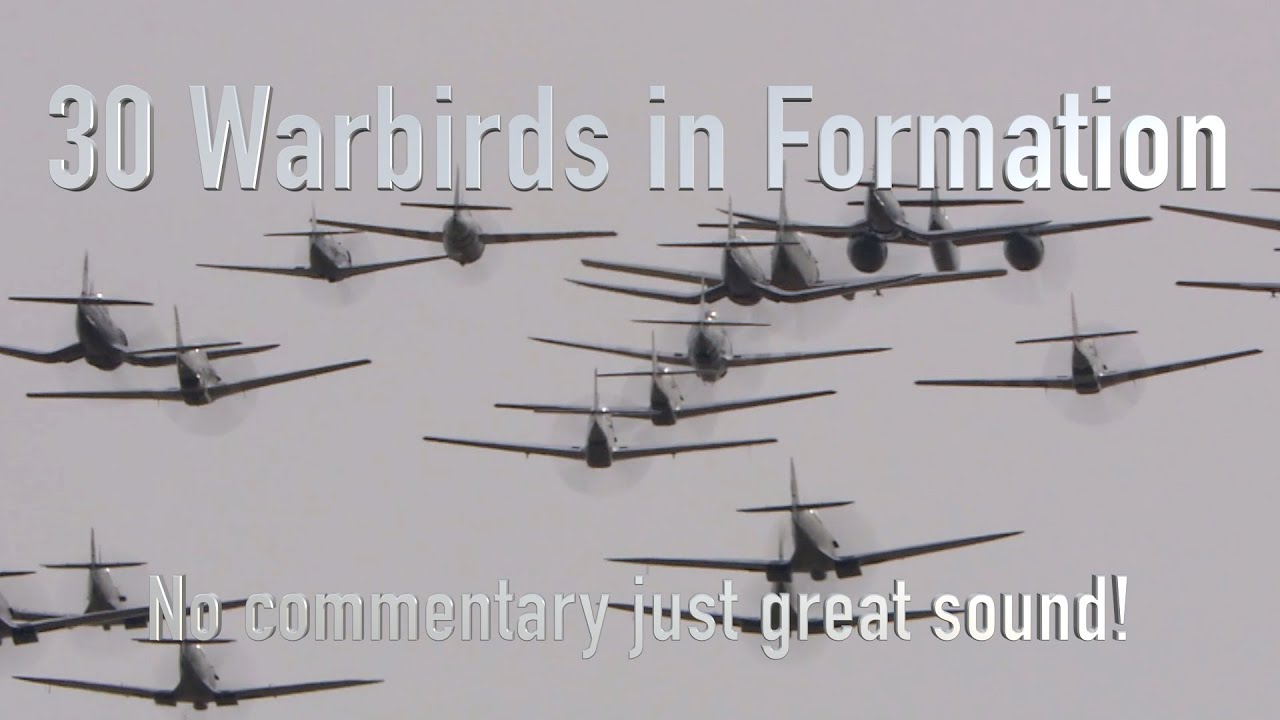This outdoor black-and-white photograph depicts a striking formation of approximately 16 single-engine World War II airplanes flying away from the camera against a somber, gray sky. The sleek, propeller-driven aircrafts are likely P-51 fighters, known for their distinctive design, and are arranged meticulously in formation, creating an impressive and historical scene. The rectangular image is augmented with overlay text: "30 warbirds in formation" boldly adorns the top, while "no commentary, just great sound" trails across the bottom. The text, starting in a silver hue and gradually transitioning to white from left to right, emphasizes the powerful and silent flight of these historical planes. The image's monochromatic tone underscores its vintage feel, combined with the ambiguity of the planes' origins, as no country markings are visible, leaving it open to interpretation.